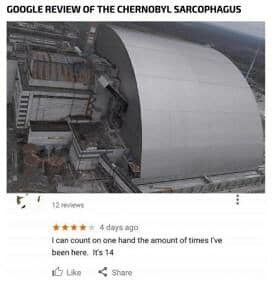This image is a dark humor meme that features a Google review of the Chernobyl Sarcophagus. The top text reads, "Google review of the Chernobyl sarcophagus," and beneath it is an aerial photograph of the infamous reactor site. The central structure is a large, grey, dome-shaped building with surrounding industrial elements such as pipes and walkways. The review section states, "12 reviews, 4 stars out of 5, 4 days ago," followed by the review that humorously notes, "I can count on one hand the amount of times I've been here. It's 14," implying radiation-induced mutation. The image is slightly blurry and lacks fine detail, but clickable "like" and "share" icons are visible below the review. Overall, the screenshot has a white background and captures the desolate and industrial expanse of the Chernobyl site, further emphasizing the morbid humor.